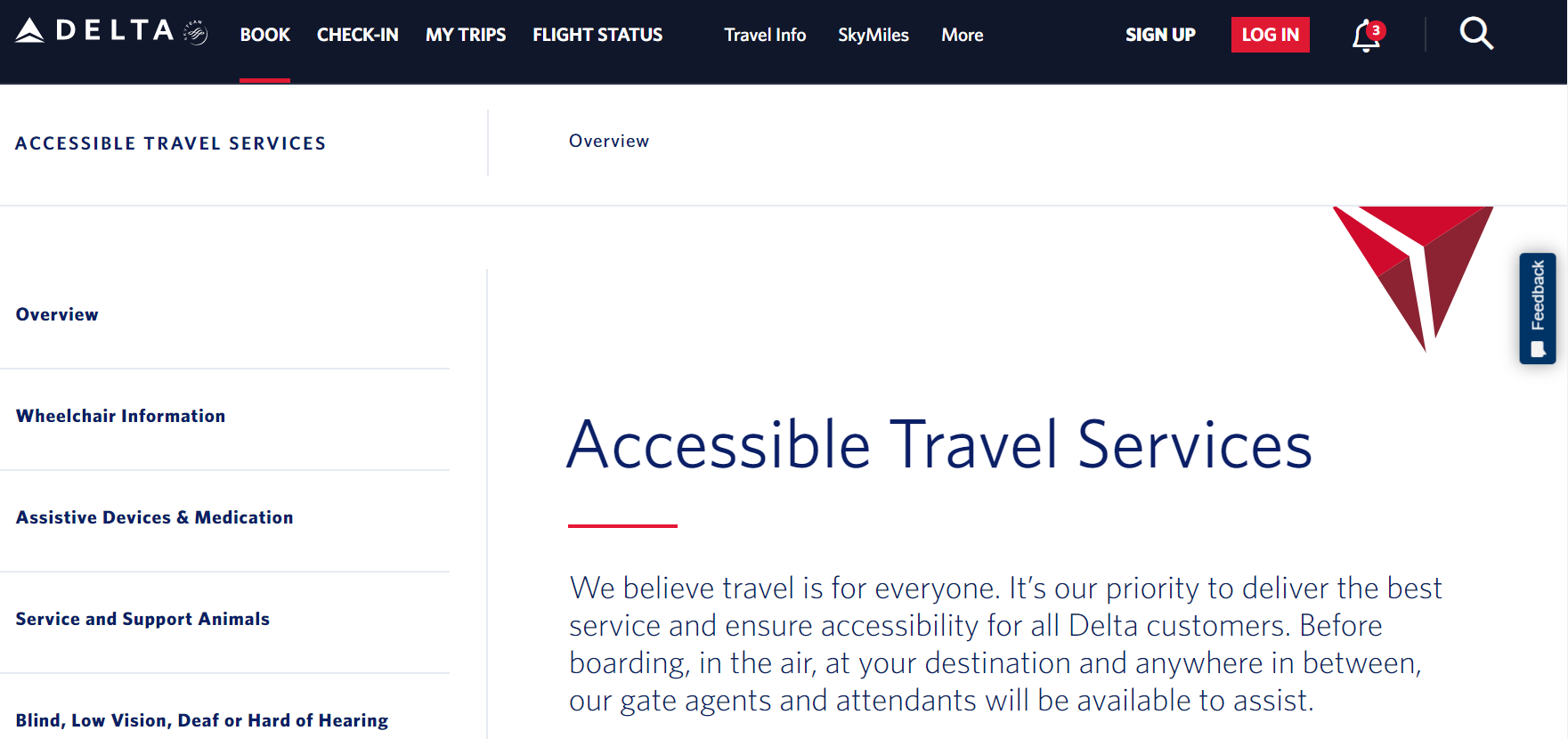The image depicts the Delta Airlines website interface. At the top left corner, the Delta logo features prominently in white text accompanied by a small triangular symbol. Directly beneath, the navigation bar includes categories such as "Book," "Check-In," "My Trips," and "Flight Status," all in white text. The "Book" category is underlined in red, indicating it is currently selected. Smaller text categories like "Travel Info" and "SkyMiles" are also present. 

On the right-hand side, options for signing up or logging in are available, with "Log In" highlighted in red. A bell icon indicating three notifications and a magnifying glass symbol for search are also situated here.

The left-hand corner of the screen displays a sidebar with blue text headings: "Accessible Travel Services," "Overview," "Wheelchair Information," "Assistive Devices and Medication," "Service and Support Animals," "Blind or Low Vision," and "Deaf or Hard of Hearing." The overview section reads: "Accessible Travel Services: We believe travel is for everyone. It is our priority to deliver the best service and ensure accessibility for all Delta customers. Before boarding, in the air, at your destination, and anywhere in between, our gate agents and attendants will be available to assist." This text is all in blue on a white background. Below the overview, a red triangular icon points to the right, and a small blue "Feedback" icon invites users to leave feedback regarding their website experience.